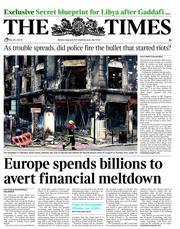The Times – Exclusive: A secret, limited edition print documenting Libya's tumultuous period after Gaddafi reveals the scene of devastation. Amid escalating unrest, questions arise whether the police fired the shot that ignited the violence. The photograph captures a smoldering, burnt-out building, now a heap of brown, gray, and black rubble, with a solitary figure standing outside. Simultaneously, Europe scrambles to invest billions in an effort to stave off financial collapse. The stark black-and-white imagery emphasizes the gravity of the situations depicted.